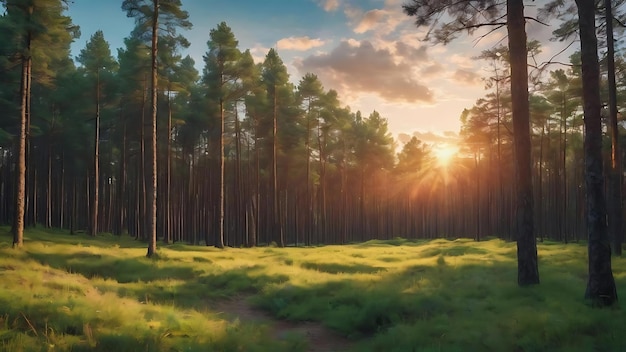This scene, which is either a photograph or a computer-generated image, captures a tranquil forest clearing with lush greenery blanketing the ground. Tall, skinny trees—appearing almost pine-like with a few leaves or needles concentrated at their tops—stand in evenly spaced rows, their long trunks rising skyward. To the left, there is a dried creek bed or dirt path cutting through the grass. As you gaze toward the horizon, the sun is either rising or setting, its yellow rays piercing through the tall tree trunks, casting a mix of sunlit and shady patches over the clearing. The sky above is a vibrant blue with fluffy white and subtle gray clouds scattered around the glowing sun, which completes the idyllic, bucolic scene.